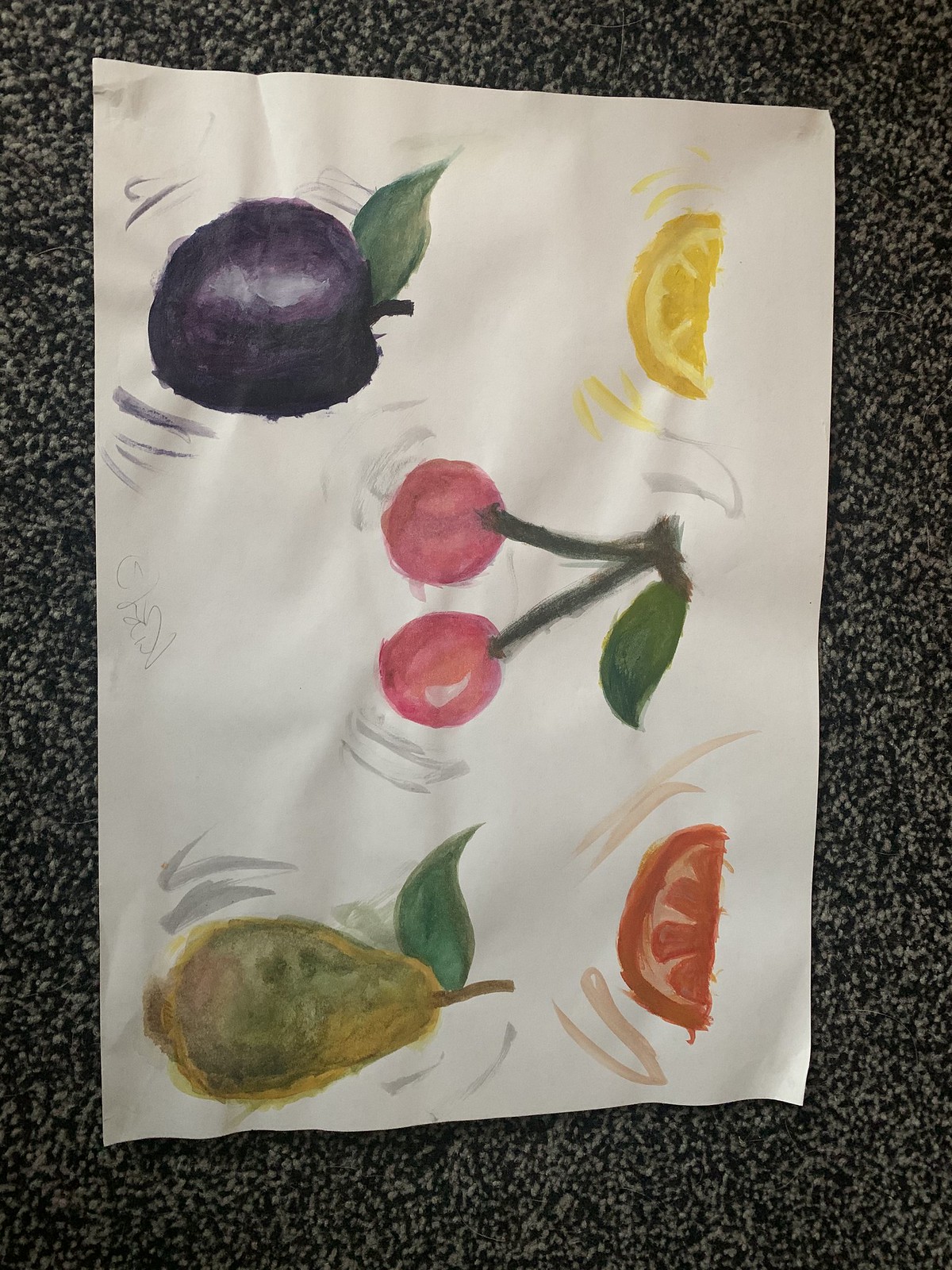A detailed and cleaned-up caption for the image could be:

"A slightly crumpled piece of white paper, possibly canvas, rests on a dense gray rug. The drawing captured on the paper features five vibrantly colored fruits: an orange, a grapefruit, a plum, a pear, and, at the center, a pair of cherries connected by a green stem. The composition is oriented sideways from the viewer's perspective, adding an abstract touch. Surrounding the fruits are dynamic gray, orange, and red streaks, giving the illusion of movement or shaking, enhancing the artwork's lively feel."